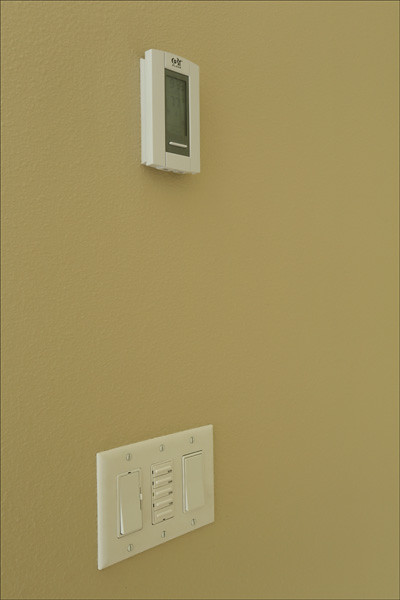The photo features a light switch positioned lower on the wall, with a modern digital thermostat mounted above it. The setup suggests a functional and contemporary climate control system for adjusting the room temperature. The light switch and thermostat appear well-integrated into the wall, highlighting a neat and organized living space. The digital display of the thermostat provides clear and easy-to-read information, contributing to the overall sleekness of the design.